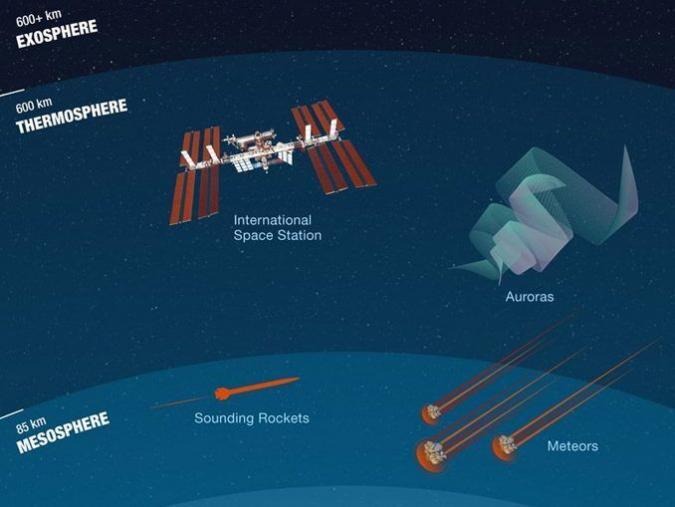The informational poster, likely from a source like NASA, illustrates different atmospheric layers and the objects found within them, using a dark-to-light blue gradient background. At the very top, the darkest region represents the exosphere, marked with "600+ KM EXOSPHERE" in white, all-caps text. Below this is the thermosphere, indicated by "600 KM THERMOSPHERE." In this zone, the International Space Station (ISS) is depicted, featuring eight rust-colored rectangular wings extending from its white central structure, with four vertical pieces. Slightly to the right of the ISS, ribbon-like, grayish-white "auroras" add detail to the thermosphere. The next layer down is the mesosphere, labeled "85 KM MESOSPHERE." This section contains an orange shooting rocket, labeled "sounding rockets," and three differently-sized meteors with faint tails, heading to the left. The poster effectively uses varying shades of blue to distinguish each layer, giving a clear and detailed representation of the different atmospheric layers and the phenomena within them.